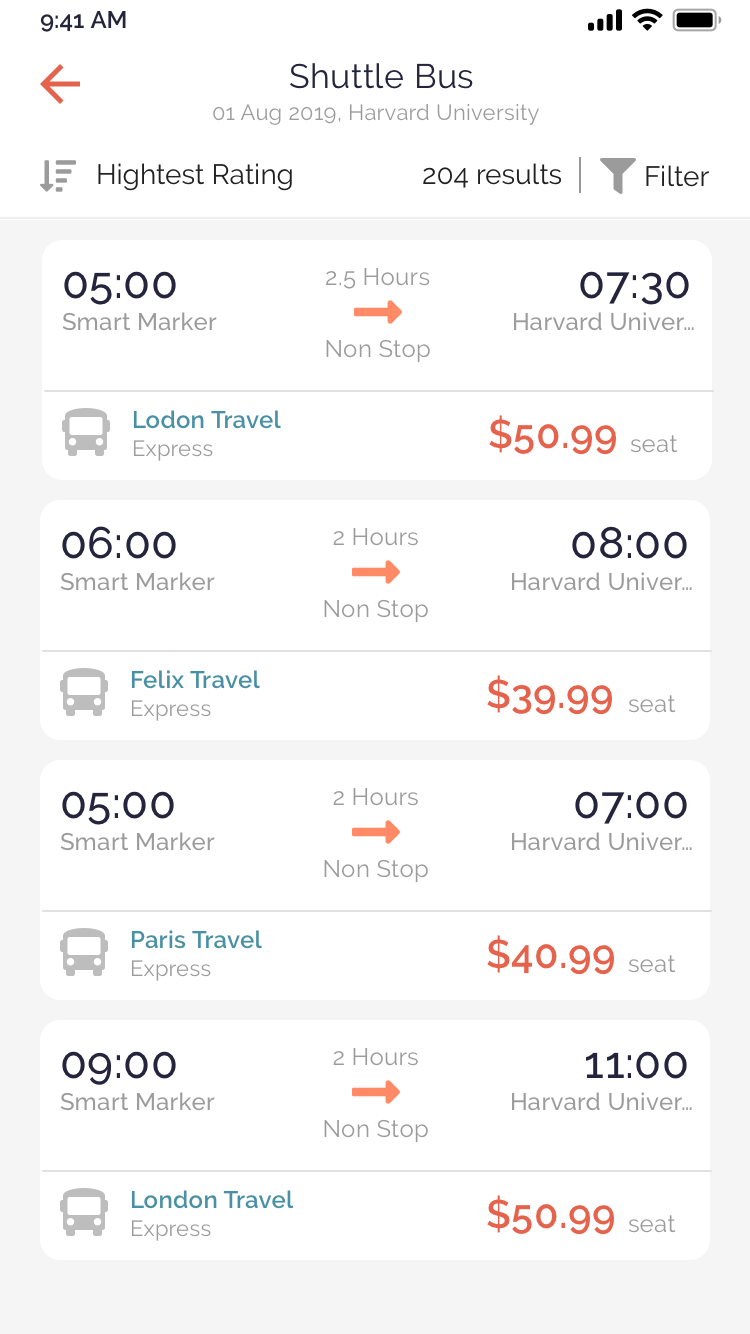A mobile screen displays detailed information about shuttle bus schedules. At the top of the screen, the status bar shows the time at 9:41 a.m., along with icons for signal strength and battery life. Below it, the heading reads "Shuttle Bus" with the date "01 August 2019" and the location "Harvard University." The screen also features an option to sort by "Highest Rating" and indicates there are "204 results" found. A filter icon is also visible for refining search results.

The first entry lists a departure time of 05:00 a.m., marked with a "Smart Marker." It details a journey of 2.5 hours nonstop, arriving at 07:30 a.m., shortened as "Harvard Univer..." A divider line separates this from subsequent entries. The next entry shows "Lodin Travel Express" with a 06:00 a.m. departure and a 2-hour nonstop journey, priced at $50.99 per seat, arriving at 08:00 a.m.

Following this, the listing for "Felix Travel" notes a fare of $39.99 per seat, with a 05:00 a.m. departure and a 2-hour nonstop trip, reaching its destination at 07:00 a.m. "Paris Travel Express" departs at 09:00 a.m. for a journey of 2 hours, costing $40.99 per seat, arriving at 11:00 a.m. The last visible entry is another from "London Travel Express," priced at $50.99 per seat, though the full details are cut off at the bottom of the screen.